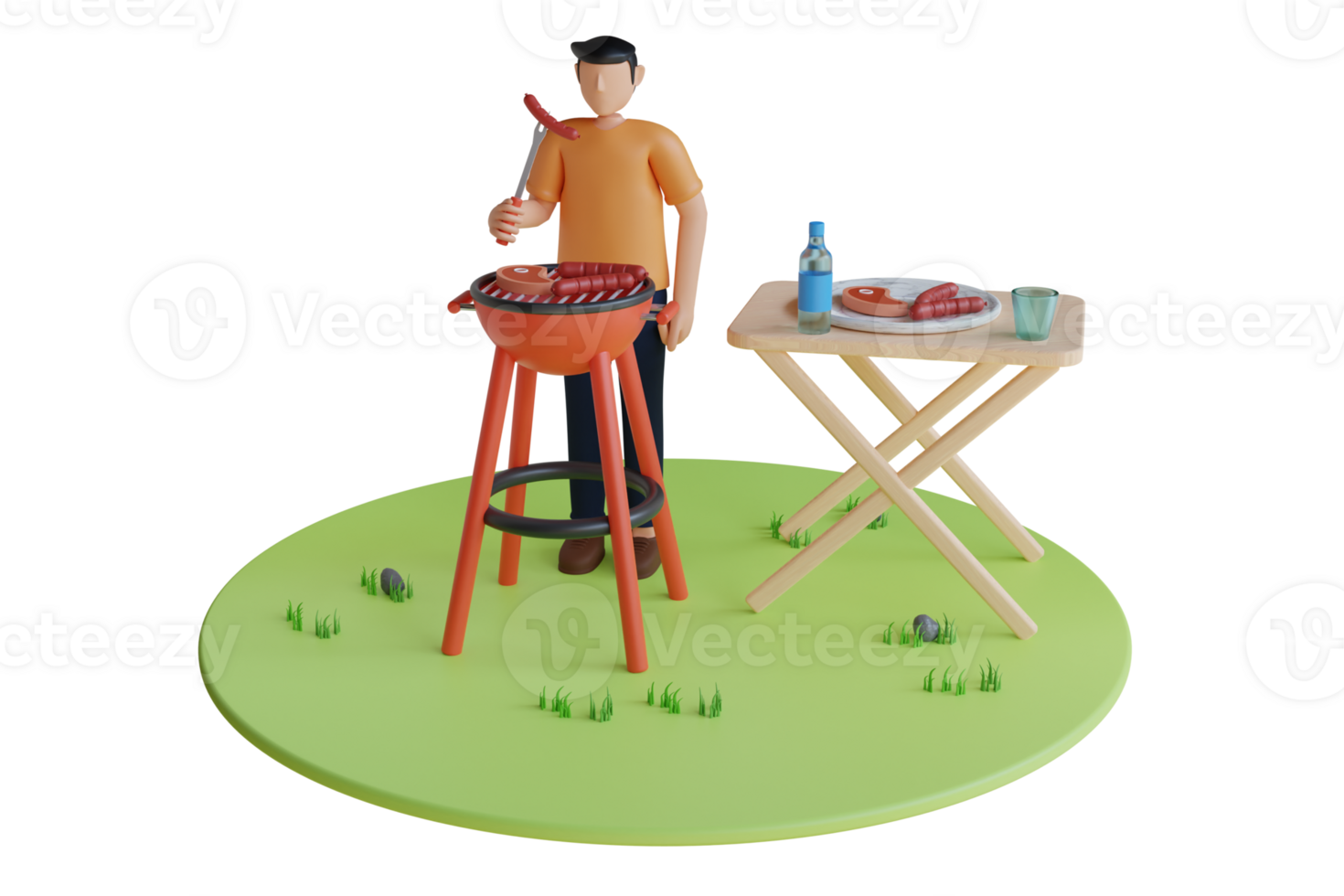This cartoon graphic from Vecteezy depicts a gentleman grilling meat on a red charcoal grill. The man, who has black hair swept to the right, is wearing an orange t-shirt, blue jeans, and brown shoes. Notably, his face is minimalistic, featuring only a nose and ears. He is standing on a circular patch of green grass with a few blades sticking up and two rocks positioned on either side of the scene.

The red grill, adorned with a black top and supported by four legs with a black ring, reaches just past the man's waist. On the grill, there are two hot dogs and a steak sizzling. In the man's right hand, he holds a long grilling fork with a hot dog skewered on it. 

To the right of the scene, positioned next to the grill, is a light tan table resembling a TV tray, which stands roughly waist-high. On the table, there is a large white plate holding two hot dogs and a steak, alongside a blue bottle (contents unspecified, possibly water or wine) and a glass. The overall image carries a lighthearted, casual vibe typical of an outdoor barbecue setting.